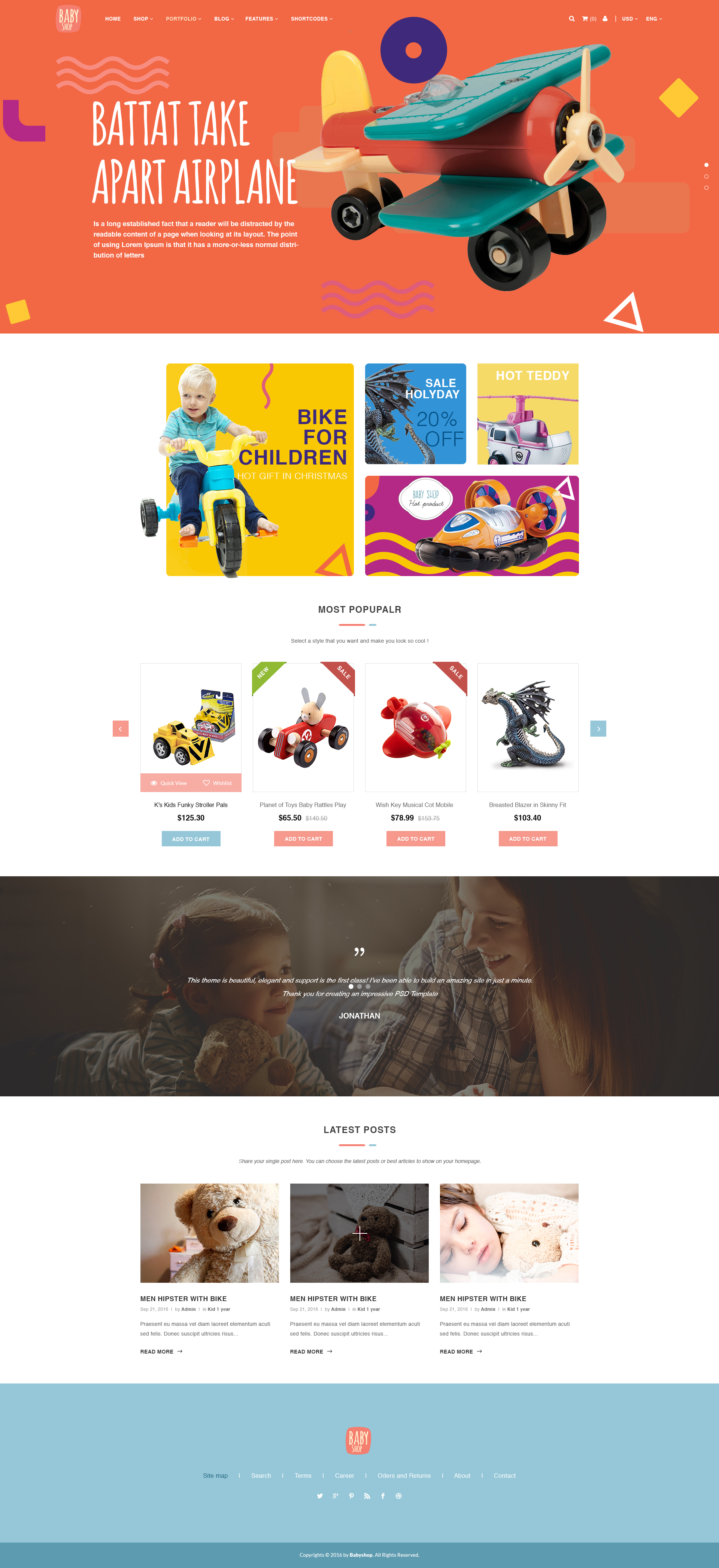This screenshot features a predominantly white background. At the top of the image is an orange rectangle with centered white, all-capitalized text reading "BAT-TAC TAKE APART AIRPLANE." To the right of this text is an illustration of a child’s wooden airplane. 

Beneath this top section are two side-by-side squares: the left square is yellow and displays an image of a child on a bike, while the right square has black text that reads "Bike for Children." 

Below these squares lies another section composed of three pictures: two side-by-side squares at the top and a single horizontally-aligned rectangle beneath them. 

Following this, there are four visible images of children's toys arranged horizontally, with navigational arrows (a blue one on the right and a red one on the left) allowing for scrolling through additional pictures.

Further down the image, there is a rectangular photograph with a dark background, depicting a child on the left and a mother on the right. This photograph is accompanied by small, unreadable white text.

Finally, the bottom section consists of three squares aligned horizontally, each containing a different image: the left square features a teddy bear, the middle one shows an ambiguous dark scene possibly involving snow, and the right square displays a sleeping woman with a dog lying on her chest. There is minimal, finely printed text situated above and below these squares. At the very bottom, a blue-green rectangle with white writing inside it concludes the screenshot.